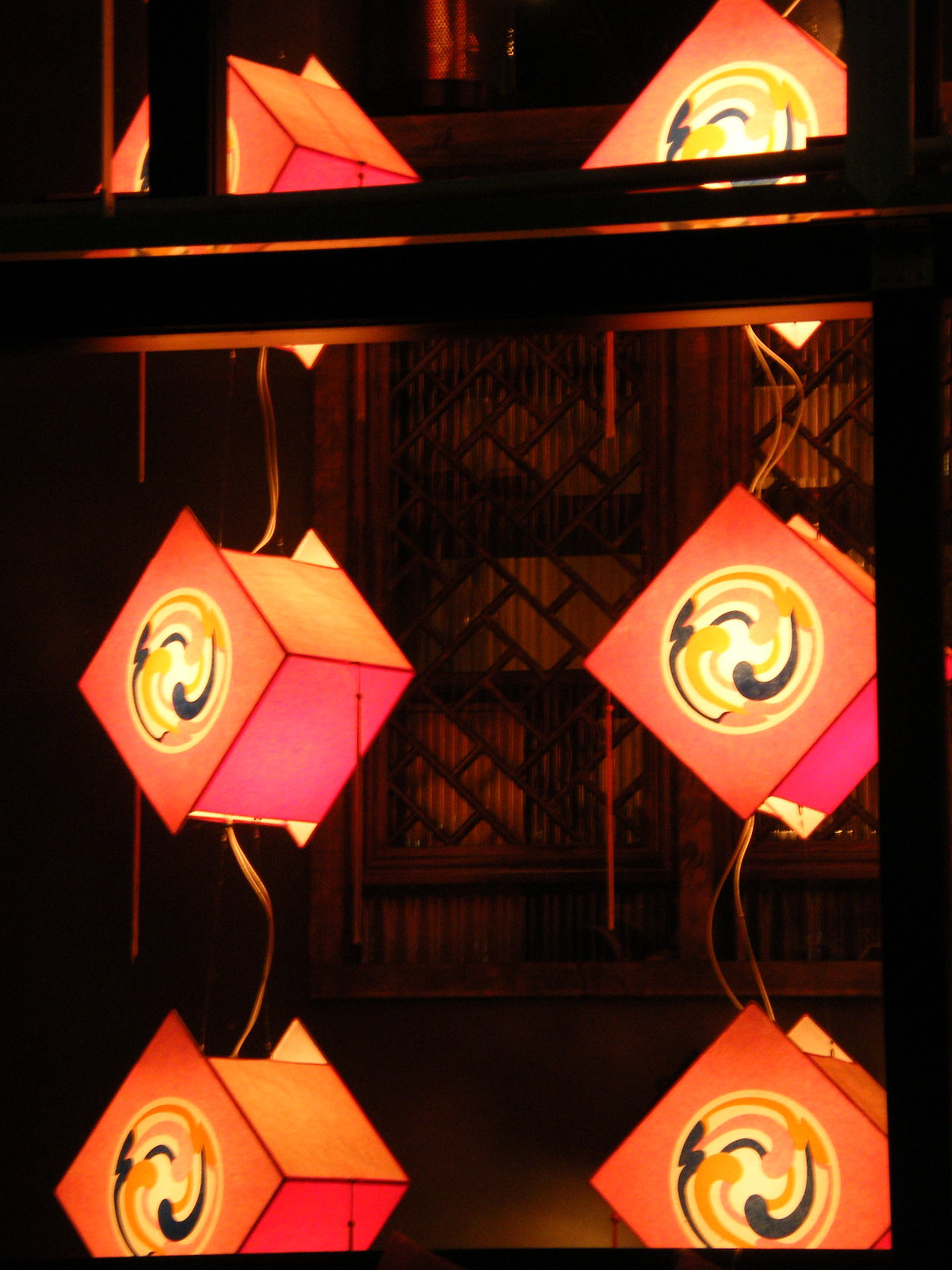In this nighttime photo, we observe a captivating display of six illuminated square lanterns, reminiscent of traditional Asian lanterns. These lanterns are suspended at a 45-degree angle from a wire, forming an eye-catching arrangement within a rack. Their vivid hot pink and orange hues are adorned with intricate gold, dark green, yellow, and black spiral designs that emit a warm, glowing light. Each lantern features red tassels hanging below, and their angular positions—tilted with points up, down, left, and right—enhance their cube-like appearance. The scene is set against a dark background with a black mesh lattice that suggests a geometric window covering, contributing to the ethereal ambiance. Foregrounding this mesh lattice work, the cords and orange strings intricately weave between the lanterns, tying the entire display together. The combination of colors and the unique arrangement offers a striking visual contrast against the dim surroundings, creating a scene that's both serene and mesmerizing.